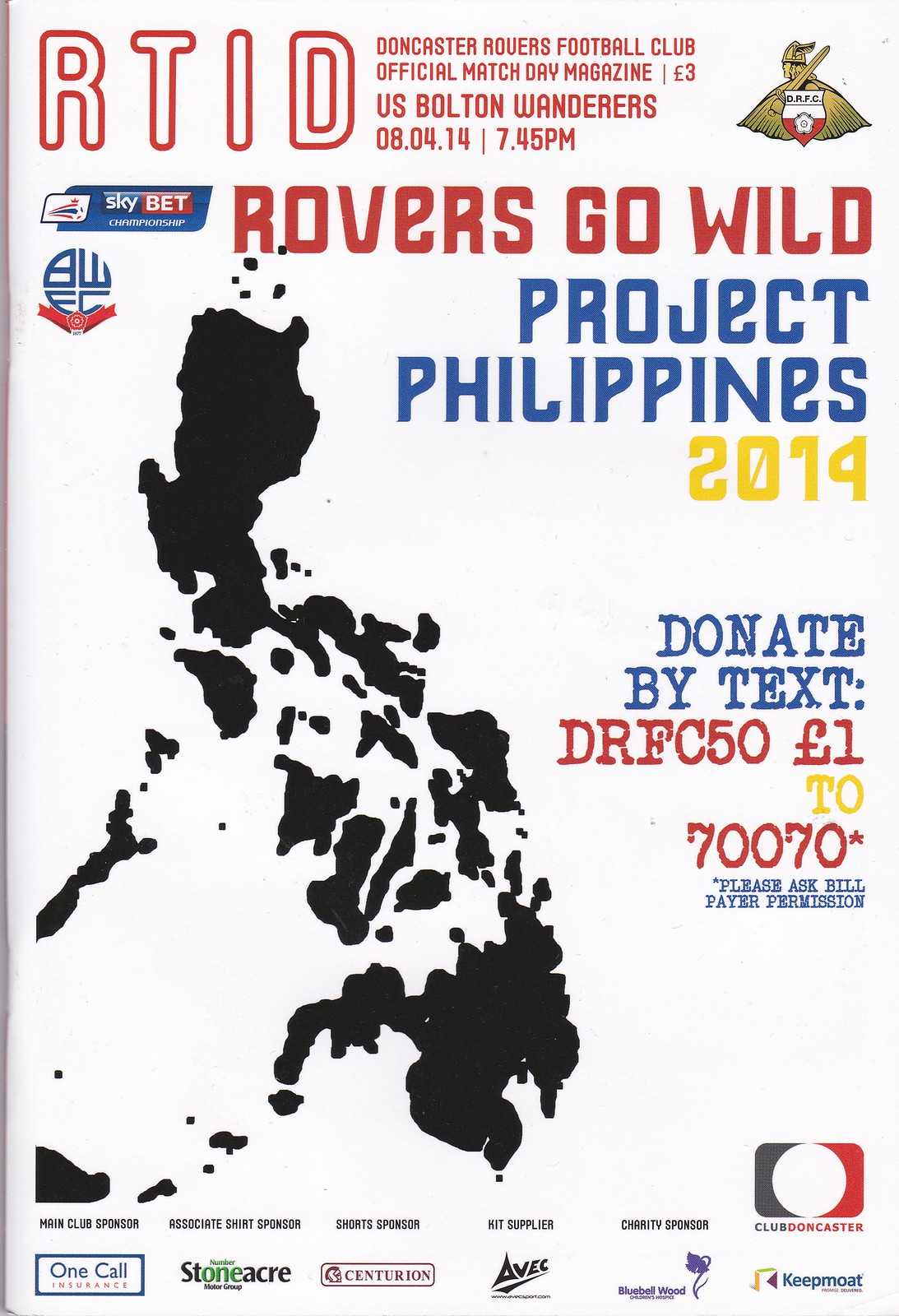This poster advertises the Doncaster Rovers Football Club's official match day magazine for a game against Bolton Wanderers on 08.04.14 at 7.45 PM, priced at three pounds. The top left corner features "RTID" in 3D all caps lettering. Centrally, the top section lists the club, match details, and the price. The club crest is located in the top right corner. Sponsors like Sky Bet Championship and WEC are displayed along the left edge, with the Sky Bet logo being particularly prominent.

In red, bold capital letters: "ROVERS GO WILD" is followed by "PROJECT PHILIPPINES 2014" in blue and yellow text. Below these slogans, a donation appeal reads: "DONATE BY TEXT: DRFC50 £1 TO 70070" and below that, in smaller blue text: "Please ask bill payer permission". 

A black silhouette of a land mass, likely representing the Philippines, with text appeals alongside it, covers much of the left side. The bottom section lists additional sponsors, featuring logos for One Call (main club sponsor), Stoneacre (associate shirt sponsor), Centurion (short sponsor), and AVEC (kit supplier). There is also a purple flower emblem for Bluebell Wood and logos for Club Doncaster and Keepmoat. The background is primarily white, giving a clean look to the various vibrant logos and text.